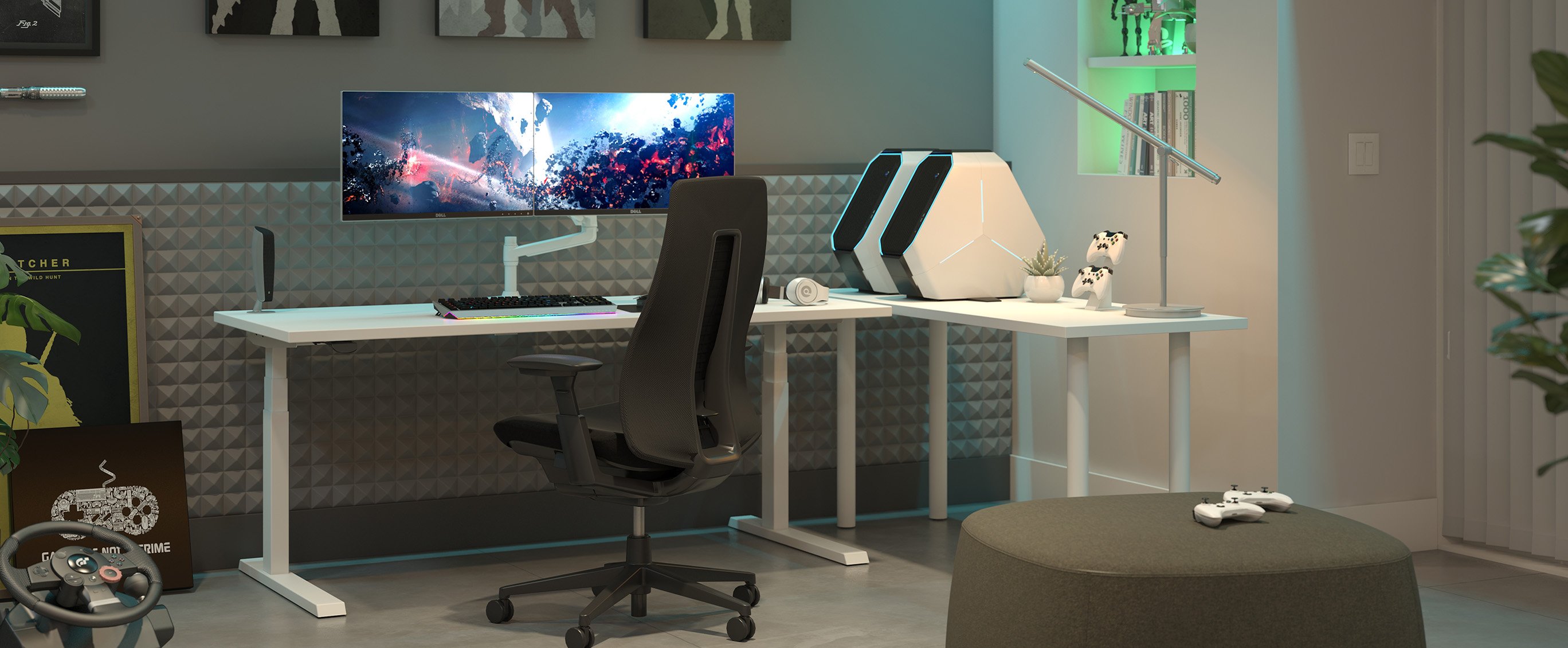The image depicts an elaborate gaming and tech-centric setup, likely situated in someone's personal room. To the left, prominently visible, is a Wi-Fi router positioned next to a dual-monitor computer setup, ensuring robust connectivity and ample screen real estate for multitasking or enhanced gaming experiences. To the right of the monitors are two units that appear to be different PCs or components thereof, suggesting a high-performance or specialized computing arrangement. Below and to the right of these units, a stand holds a pair of Xbox controllers, emphasizing the gaming focus of the space. In the bottom left corner of the photo, a steering wheel controller designed for racing games can be seen, further hinting at the room's use for various gaming activities. Overall, the room is meticulously arranged to accommodate both gaming and technological pursuits, manifesting a dedicated personal gaming and tech sanctuary.